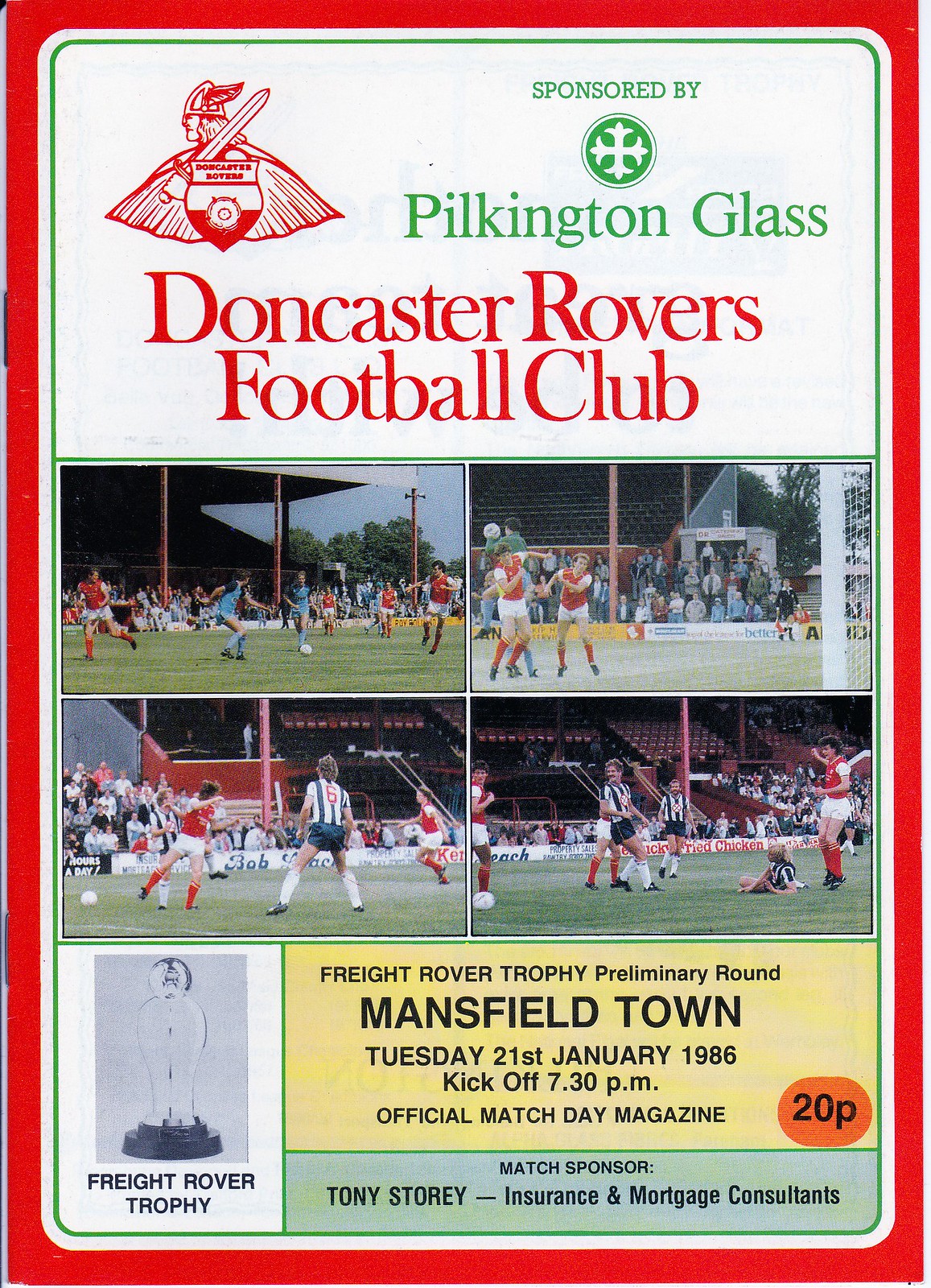**Detailed Caption:**

The image depicts a promotional cover for the Doncaster Rovers Football Club. At the top, the club's sponsor, Silky Pink Glass, is prominently displayed. The main body of the image features Doncaster Rovers in their traditional red kits, with the sponsorship details highlighted in green. Central to the design is the club's emblem, which is depicted as a red knight or Viking figure.

The cover is segmented into four images illustrating the team actively playing football, with scenes showing players running across the field and the presence of a referee. 

At the bottom of the cover, the text reads:
"Freight Rover Trophy Preliminary Round, Mansfield Town, Tuesday, 21st January 1986, kickoff 7:30 PM, official Match Day magazine, 20 pence."

Additionally, the bottom section identifies the sponsor, Tony Story Insurance and Mortgage Consultants, and displays the logo and name "Freight Rover Trophy" accompanied by an image of the trophy.